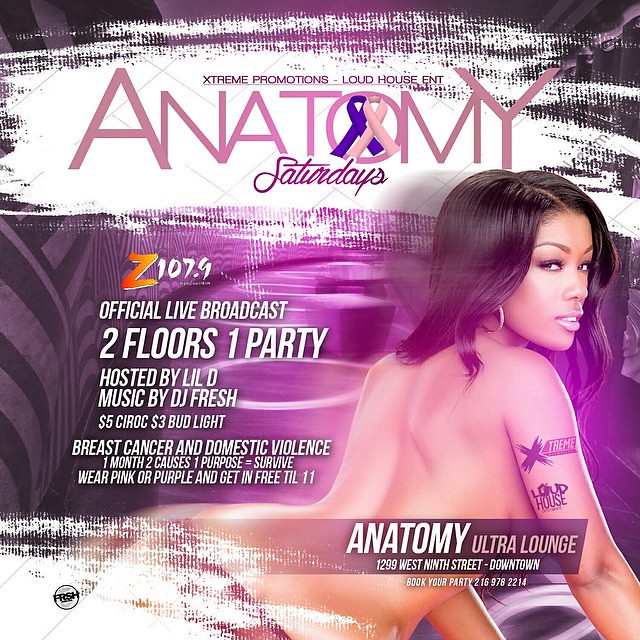The image is an advertisement for a party event at the Anatomy Ultra Lounge, located at 1299 West 9th Street, Downtown. The background features various shades of purple with swirls and different patterns, accented by a white, rubbed-in area on the upper right that displays "Extreme Productions," "Loud House ENT," and "Pink Anatomy Saturdays." 

In the upper portion, white text announces an official live broadcast by Z107.9, indicating "Two Floors, One Party," hosted by Lil D with music by DJ Fresh. Additionally, the advertisement promotes special offers, including $5 Ciroc and $3 Bud Light, and encourages guests to support breast cancer and domestic violence awareness by wearing pink or purple to gain free entry until 11 PM.

The lower half of the image features an African-American woman with shoulder-length hair and an earring posed suggestively, facing the camera while leaning to the right. Her private parts are tastefully covered by additional banners and text. Notably, she has a tattoo that reads "Extreme" and "Loud House." The ad encourages viewers to book their parties at this location by providing a phone number for reservations. 

Overall, the vivid colors of black, pink, purple, tan, white, gray, orange, and yellow create a vibrant and eye-catching design, emphasizing the nightclub's festive and energetic atmosphere.